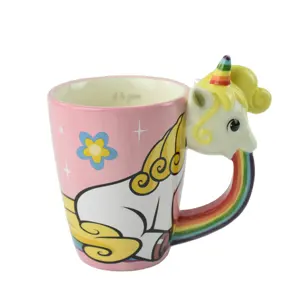In this detailed product photograph of a ceramic coffee mug, the background is transparent, likely indicating it's intended for online sale. The main body of the mug features a whimsical design with a pink background adorned with white stars and blue flowers each with a yellow center. The central attraction is the depiction of a unicorn, characterized by its white body, yellow mane, and yellow tail. The unicorn appears to be sitting down, seamlessly integrated into the design.

The most striking feature, however, is the mug's handle. Protruding from the right-hand side of the mug is the three-dimensional head of a unicorn with a white face, yellow mane, and a rainbow-colored horn. From the unicorn's mouth, a rainbow arc extends downward, forming the curved handle of the mug. This rainbow is vividly colored in red, orange, yellow, green, blue, and dark purple. The interior of the mug is white, contrasting with the colorful and imaginative exterior. All elements combine to create a playful and visually engaging product, emphasizing the unicorn theme with a touch of magical charm.